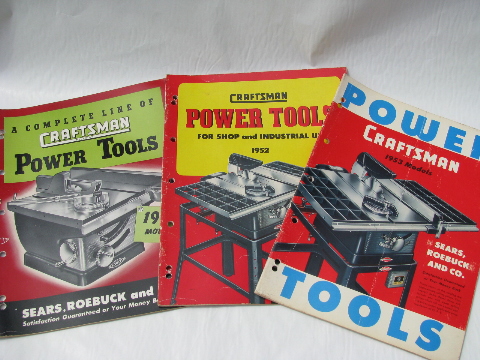This detailed photograph showcases three vintage Sears Roebuck catalogs, each primarily promoting Craftsman power tools from the early 1950s. 

The catalog on the left features a vivid green and red background, prominently displaying a table saw on its cover. It reads "A complete line of Craftsman power tools" at the top within a green box and "Sears, Roebuck and Co." along with “Satisfaction guaranteed or your money back,” partially obscured by the overlapping middle catalog.

The central catalog, dated at 1952, is adorned with a red background and a yellow rectangle stating "Craftsman power tools for shop and industrial use." The image depicts a table saw, emphasizing the industrial application of the tools.

The catalog on the right, bearing the date 1953, also carries a red background with two white bands at the top and bottom. The top reads "Power" and the bottom "Tools," both in a striking blue font. Within the white bands, it is labeled "Craftsman 1953 models" and features a table saw prominently displayed in the center. The text also identifies "by Sears, Roebuck and Co."

All three catalogs are set against a white background, likely a sheet, and slightly overlap each other, creating a cohesive and nostalgic snapshot of mid-20th-century Craftsman tool marketing.